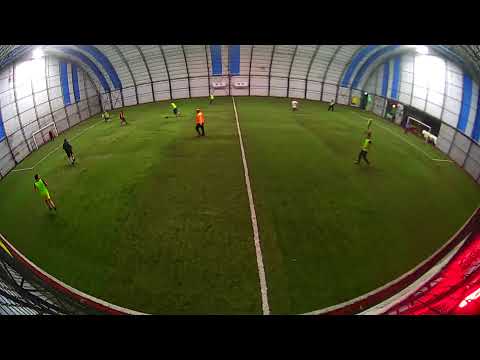This photograph captures an indoor soccer game in full action. The image, horizontally aligned and framed by thick black borders at the top and bottom, offers a fisheye perspective that emphasizes the field’s dome-shaped, hangar-like structure. The field itself is green turf, bisected by a prominent vertical white line that divides it into two halves. Goalposts are stationed at either end of the field, guarded by vigilant goalkeepers.

The roof and walls of this spacious indoor arena are adorned in white and blue colors. The players on the field are dressed in various uniforms: several don neon green vests while others sport white and black tops, and an individual in an orange shirt, likely the referee, stands centrally. Despite the players being some distance away, the elevated vantage point suggests the photo could have been taken from a high position, perhaps the stands, creating a comprehensive view of the scene. The background hints at some structural elements and a doorway or walkway, adding to the sense of a large, enclosed space where artificial lights softly illuminate the playing area, highlighting the energetic atmosphere of the indoor soccer game.